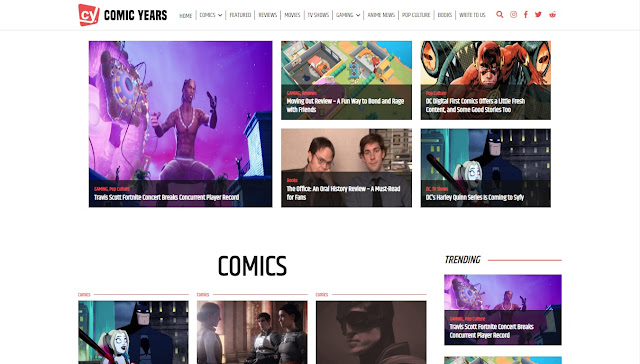The screenshot is from the Comic Years website. At the top, the header features a red box with the letters "CY" in white, and next to it "Comic Years" in black text. This is followed by a navigation bar with options such as Home, Comics, Featured, and Reviews, accompanied by icons for Facebook, Twitter, and a red magnifying glass indicating a search feature. 

In the main content area, the top left showcases an image of Travis Scott at a concert, which is identical to a smaller image in the Trending section on the right. Below the header are several image panels displaying various articles: one featuring characters from the TV show "The Office," another related to Batman and Harley Quinn, an article with the Flash, and another about The Sims. 

The next section labeled "Comics" in bold black letters displays three article previews: one featuring Batman, another with a woman talking to two boys, and a third showing a black-and-white image of a man. To the right, the Trending section is marked with black letters and a red line, featuring additional images, including the one of Travis Scott.